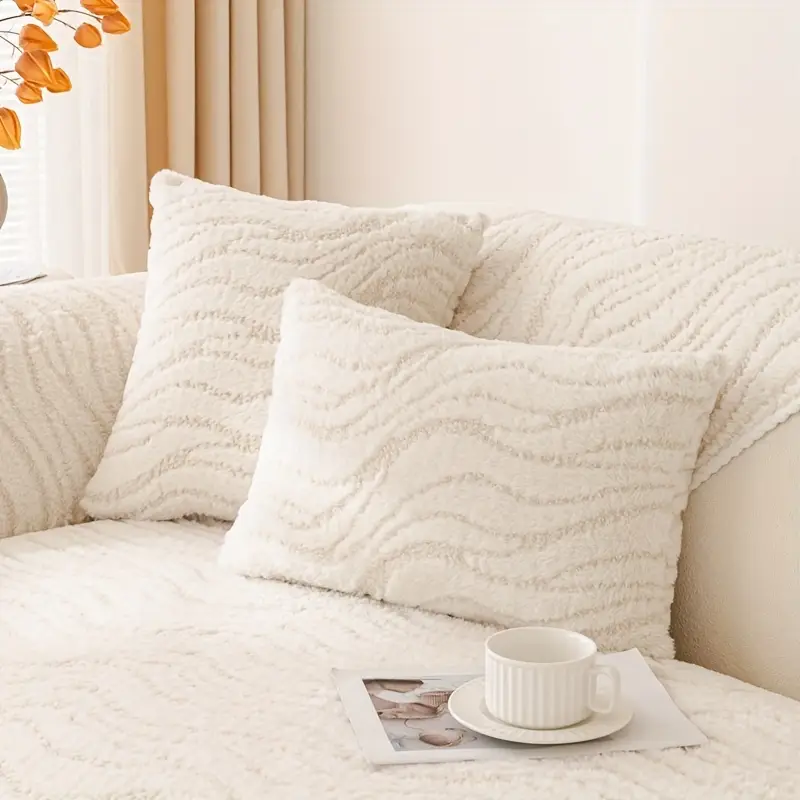This detailed close-up image captures the corner section of a white fabric couch adorned with two pillows featuring gray and white zebra stripes. A neatly folded matching blanket rests in the corner of the couch. On the seat, a stylish vignette includes a coffee cup on a saucer placed atop a magazine, contributing to a cozy, lived-in feel. The background displays a cream-colored wall occupying the upper two-thirds of the image, complemented by peach and white curtains with vertical slats on the left side. Additionally, half a vase with vibrant orange flowers emerges from the upper left corner, enhancing the room's inviting and warm aesthetic.